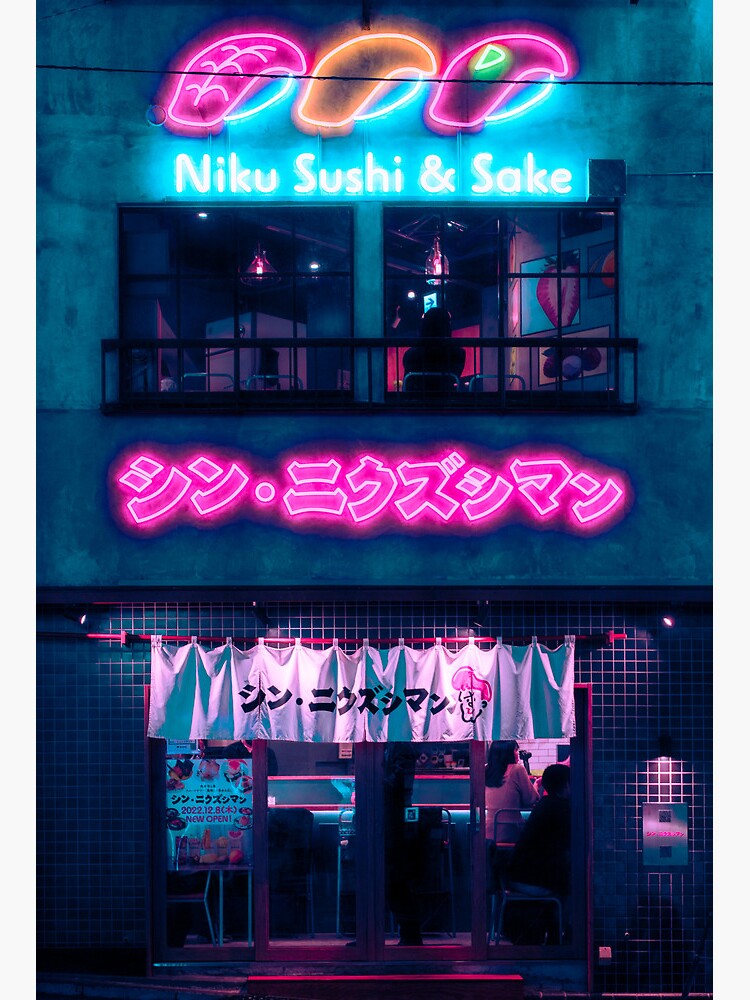This vibrant image captures the front of a two-story sushi restaurant, adorned with lively neon signs and detailed décor. The lower level features a large, turquoise drape with Japanese characters, which also displays an illustration of a person with pink hair. The entranceway is illuminated, bordered by a mix of white and pink neon lighting, creating an inviting glow. There's also a keypad on the right side and a food sign on the left. Central to the lower facade, a striking pink neon sign with Japanese script casts a rosy hue over the entire scene, further enhancing the ambiance.

The upper level of the restaurant showcases the name "Niku Sushi and Saki" in bright blue neon letters. Above this, three neon illustrations of sushi pieces in various colors – red, orange, and another red with a small green dot hinting at wasabi – add a playful touch. Visible on this level are also elements such as a balcony and a window, suggesting additional seating or dining space inside. A person stands in front of the glass entrance, appearing ready to step inside and enjoy the culinary delights the restaurant offers.